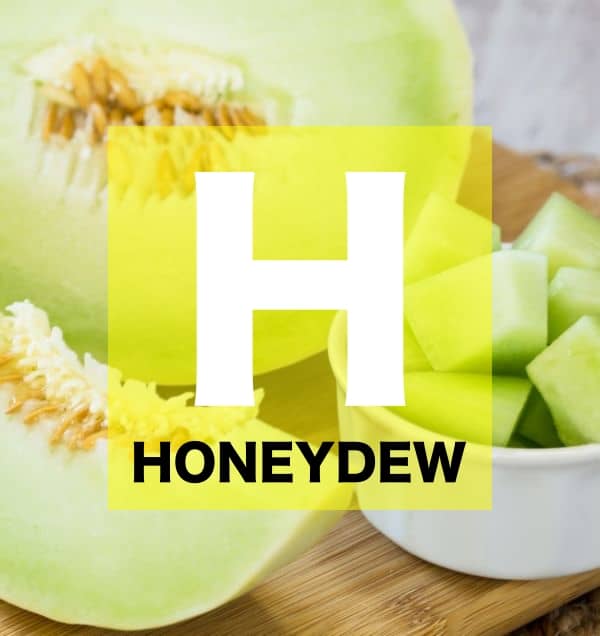This is an almost square, bright image showcasing various parts of a honeydew melon. Central to the image is a large, transparent yellow square with a prominent white 'H' at its center and the word "HONEYDEW" in black capital letters beneath it. This central element does not obscure the background details, which features a close-up arrangement of the honeydew melon and occupies a significant portion of the image. 

In the background, you see a light brown, wood-grained table with different sections of honeydew melon. On the left, there's a half-cut honeydew melon, revealing its light green interior and brown and white seeds. Adjacent to it lies a smaller eighth section of the melon, also displaying its seeds. To the right, a white bowl containing neatly chopped square pieces of honeydew melon is partially cut off by the image border. The overall composition is set against a kitchen countertop, with a soothing yet vibrant palette of yellows and greens that highlights the freshness of the honeydew melon.